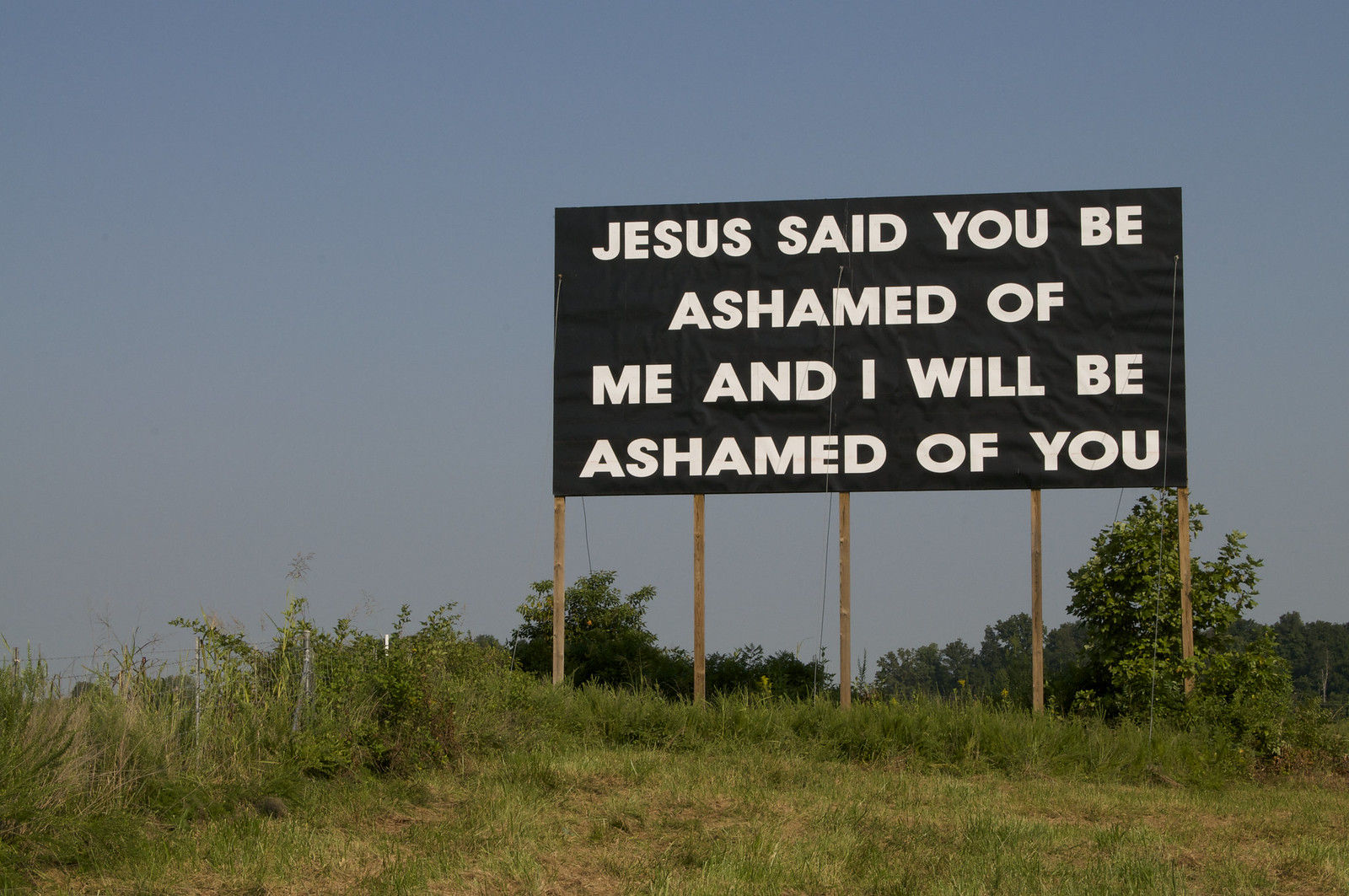In the image, a vast field of dry, brown, and green grass stretches across the foreground, creating a stark, arid landscape. Rising from this field are five wooden poles, connected by electrical wires that extend towards the back of the scene. Dominating the middle ground is a large, black billboard with white text that reads, "Jesus said, 'If you are ashamed of me, I will be ashamed of you.'" This prominent sign is situated by the side of a road. In the background, a line of trees with green leaves stands tall, contrasting with the dry grass below. A small section of a barbed wire fence is visible in the bottom left corner, further emphasizing the rural setting under a vast, open sky.